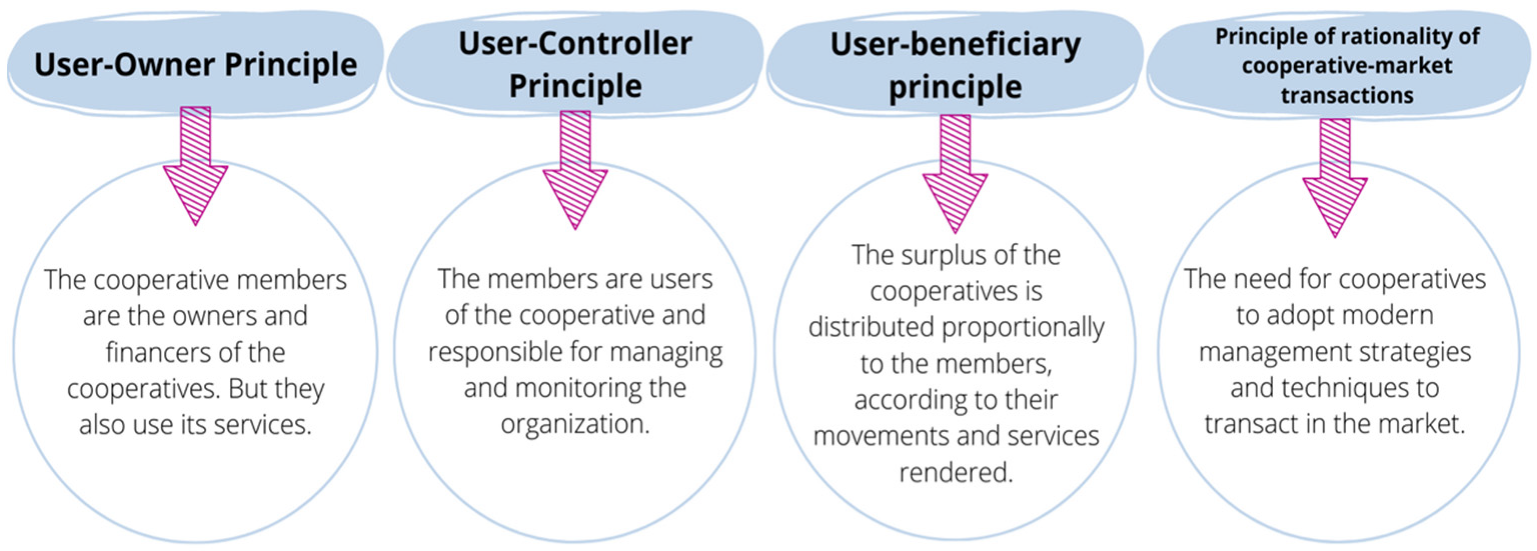The image is a detailed flowchart consisting of two rows. The top row features four oval-shaped figures with text, while the bottom row has corresponding blue-bordered circles with additional text and arrows connecting the ovals to the circles below them. Each section details specific principles related to cooperative management and operation.

The first oval, labeled "User-Owner Principle," has an arrow pointing to a circle that explains how cooperative members are both the owners and financers, utilizing the services offered by the cooperative. The second oval, "User-Controller Principle," points to a circle that emphasizes the role of members in managing and monitoring the organization. The third oval, titled "User-Beneficiary Principle," directs to a circle that outlines the distribution of surplus among members proportionally based on their activities and services rendered. The fourth oval, "Principle of Rationality of Cooperative Market Transactions," points to a circle that highlights the necessity for cooperatives to adopt modern management strategies and techniques to effectively engage in market transactions.

Overall, this flowchart visually represents the interconnected principles of cooperative ownership, control, benefit distribution, and market rationality, providing a clear overview of how cooperatives function and are managed.